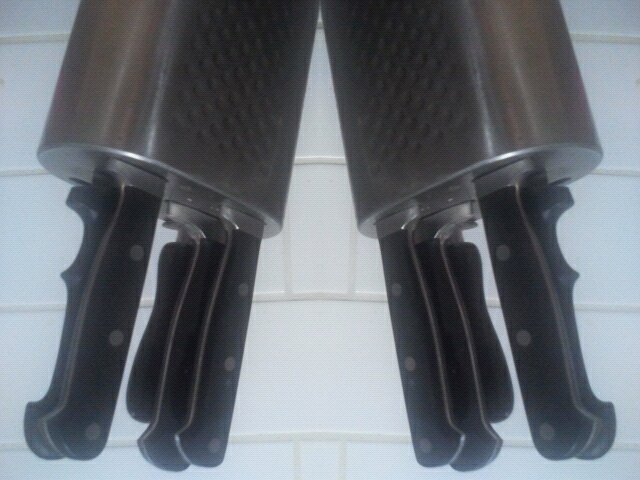The image is an upside-down photograph of two knife blocks set against a white subway tile backsplash, typical of a kitchen environment. These stainless steel knife blocks, positioned at a diagonal angle from the top center of the frame, each hold five kitchen knives. The knives are oriented with their black handles pointing downward and feature three silver rivets on each handle. The blades are inserted into slots on the metal blocks, and each block appears to mirror the other, suggesting a symmetrical design. The left block's knives are angled towards the bottom left of the photo, while the right block's knives angle towards the bottom right. The entire setup appears to be part of a professional kitchen or catering setting, consistent with the practical need for multiple sets of chef's knives.